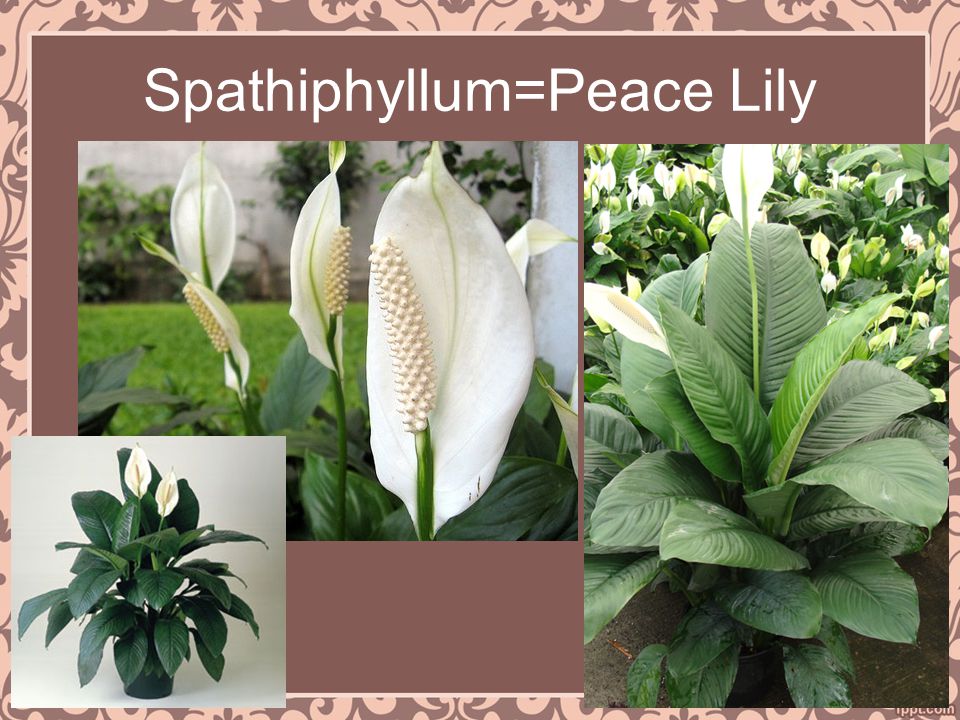This image appears to be part of an educational or presentation slide, likely designed to illustrate information about the Peace Lily, also known as Spathiphyllum. The background features a pinkish-brown hue with a light pinkish cream scrolling floral border, reinforcing its thematic aesthetic. At the top, the text "Spathiphyllum equals Peace Lily" is clearly displayed, indicating both the scientific and common names of the plant.

Within this bordered area, multiple images of Peace Lilies are scattered, with some overlapping. In the bottom left corner, a full photograph of a Peace Lily in a pot shows vibrant green leaves and two characteristic white blooms, each displaying a large petal with a central spadix. Directly above this image, there is a detailed close-up of the plant’s foliage, highlighting the healthy, unblemished green leaves. To the right, another close-up focuses on two blooms with additional lilies in the background.

The overall arrangement of the images and the descriptive text suggests that this visual is intended for educational purposes, perhaps part of a PowerPoint presentation or an informational pamphlet aimed at plant enthusiasts or students.